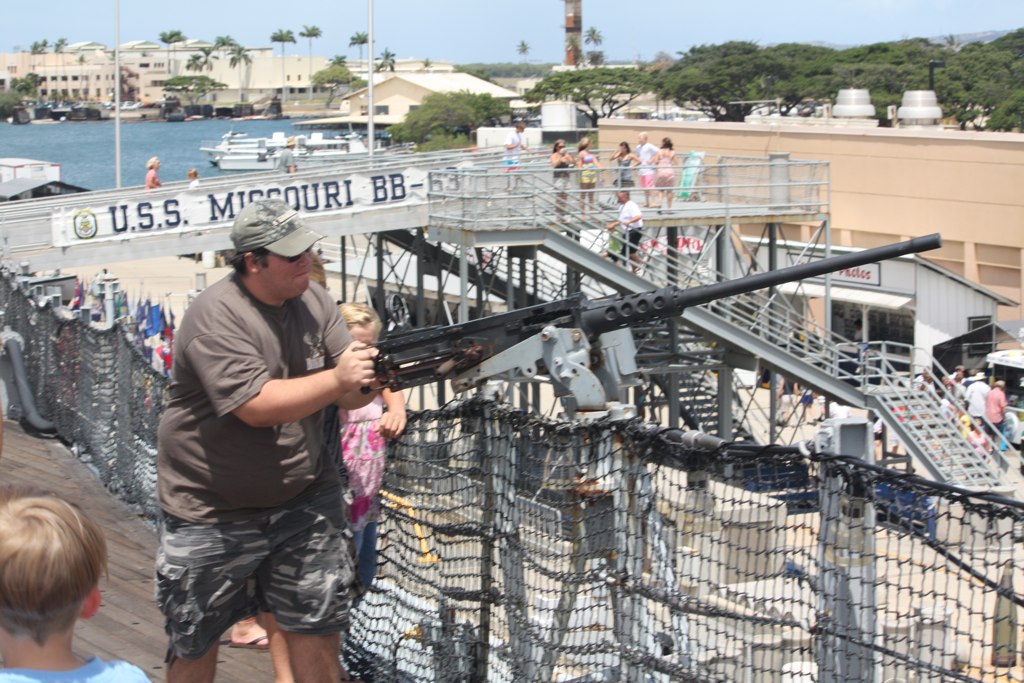The photograph captures a lively scene featuring a man interacting with a prop-style machine gun, situated on a dock rather than a battleship. The man appears to be playfully aiming the gun, which is mounted on a grayish chain-link fence, surrounded by tourists. He is dressed in camouflage cargo shorts, a gray t-shirt, and a greenish hat. To his right, one child, dressed in a pink floral dress and jeans, stands partially obscured, while another child’s head is visible in the lower left corner of the frame.

Behind the man, a large white banner reading "USS Missouri BB-63" signifies the location, potentially a naval museum or a battleship display area designated for tourists. The wooden dock-style flooring beneath the man’s feet enhances the nautical theme. In the background, several people are walking along a bridge-like structure, and five or six individuals are visible near a balcony area to the right. The setting is brightened by a clear blue sky, dotted with palm trees and other taller trees in the distance, along with a view of calm water featuring a few smaller boats.